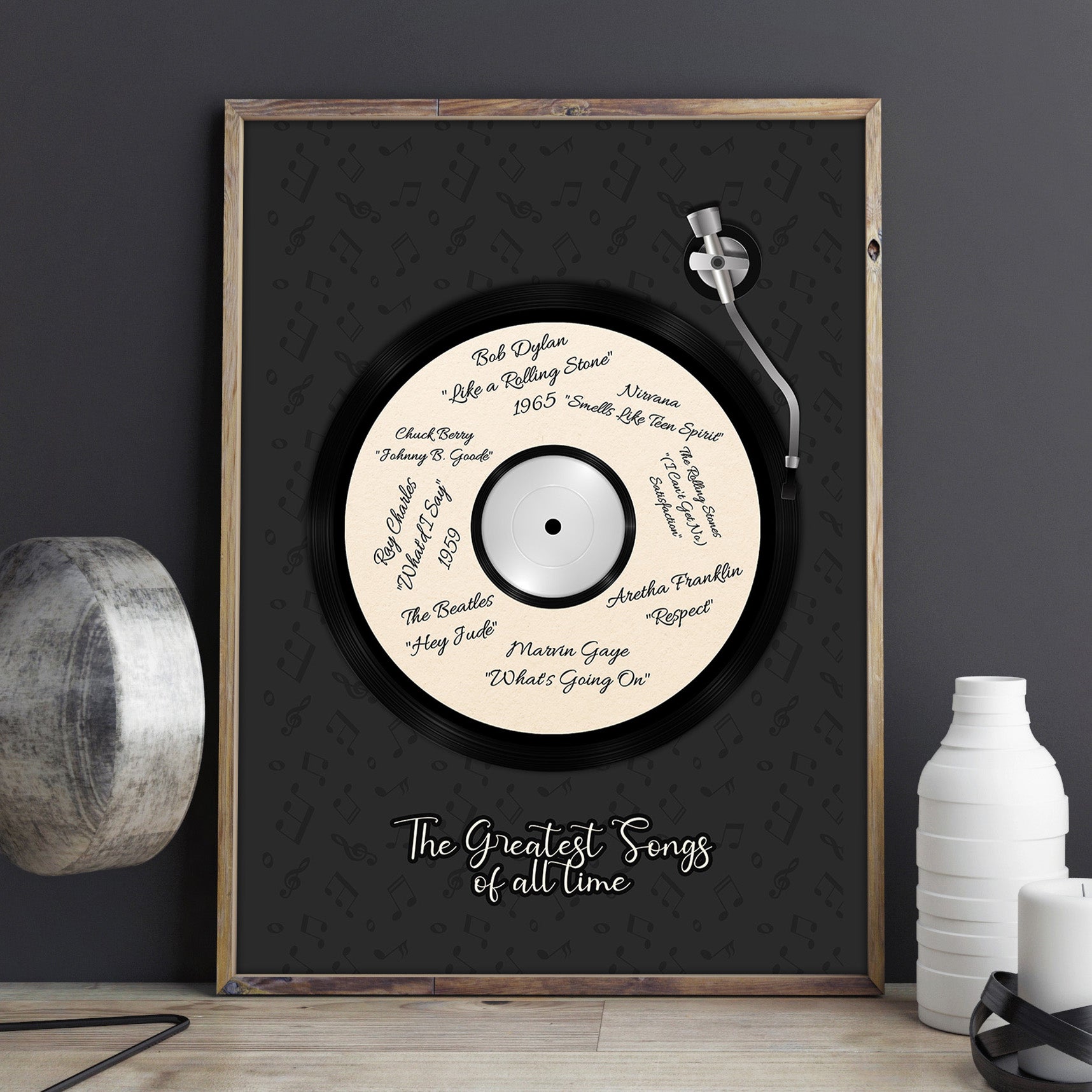The image features a framed CD presented as an award for "The Greatest Songs of All Time," prominently displaying this phrase in white script. The CD itself is white with various legendary song titles, including Bob Dylan's "Like a Rolling Stone," Nirvana's "Smells Like Teen Spirit," Marvin Gaye's "What's Going On?" alongside names like The Rolling Stones, Chuck Berry, Ray Charles, The Beatles, and Aretha Franklin, encircling the disc. The frame, which has a wooden texture, is propped up against a grayish-colored wall on a wooden surface. To the right of the frame is an unlit white candle, adorned with a dark ribbon at its base, and a white plastic bottle without a cap. A metallic object resembling a turntable arm appears near the top right of the frame, contributing to a musical theme. Additional metal disc elements decorate the left side, completing the ensemble of items on display. The background features musical notes on a black backdrop, emphasizing the musical essence of the framed piece.